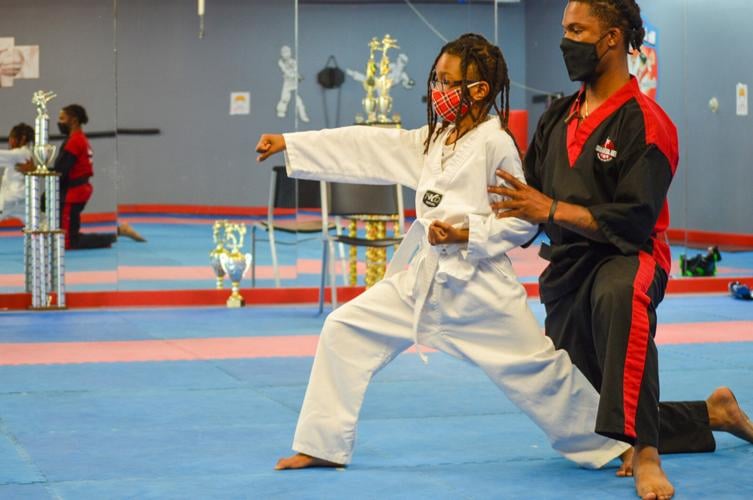The image is taken indoors in a karate dojo. In the foreground, a young Black boy with braids is practicing his karate stance on a blue mat accented with a red stripe. He is dressed in a white gi with a white belt and is barefoot, wearing glasses and a red plaid face mask. The boy's left arm is pulled back by his rib, and his right arm is extended forward, demonstrating a punch. Behind him, a Black man—presumably the instructor—kneels, guiding the boy's form with his left hand supporting the boy's left arm. The instructor is wearing a black mask along with a black and red gi. In the background, a mirrored wall reflects the pair, enhancing the sense of space within the studio. Several trophies are lined up against the mirror, and the walls of the dojo are gray with a red baseboard. The mirrored surface captures the focused expressions and the detailed posture of both teacher and student, emphasizing the discipline and instruction taking place.